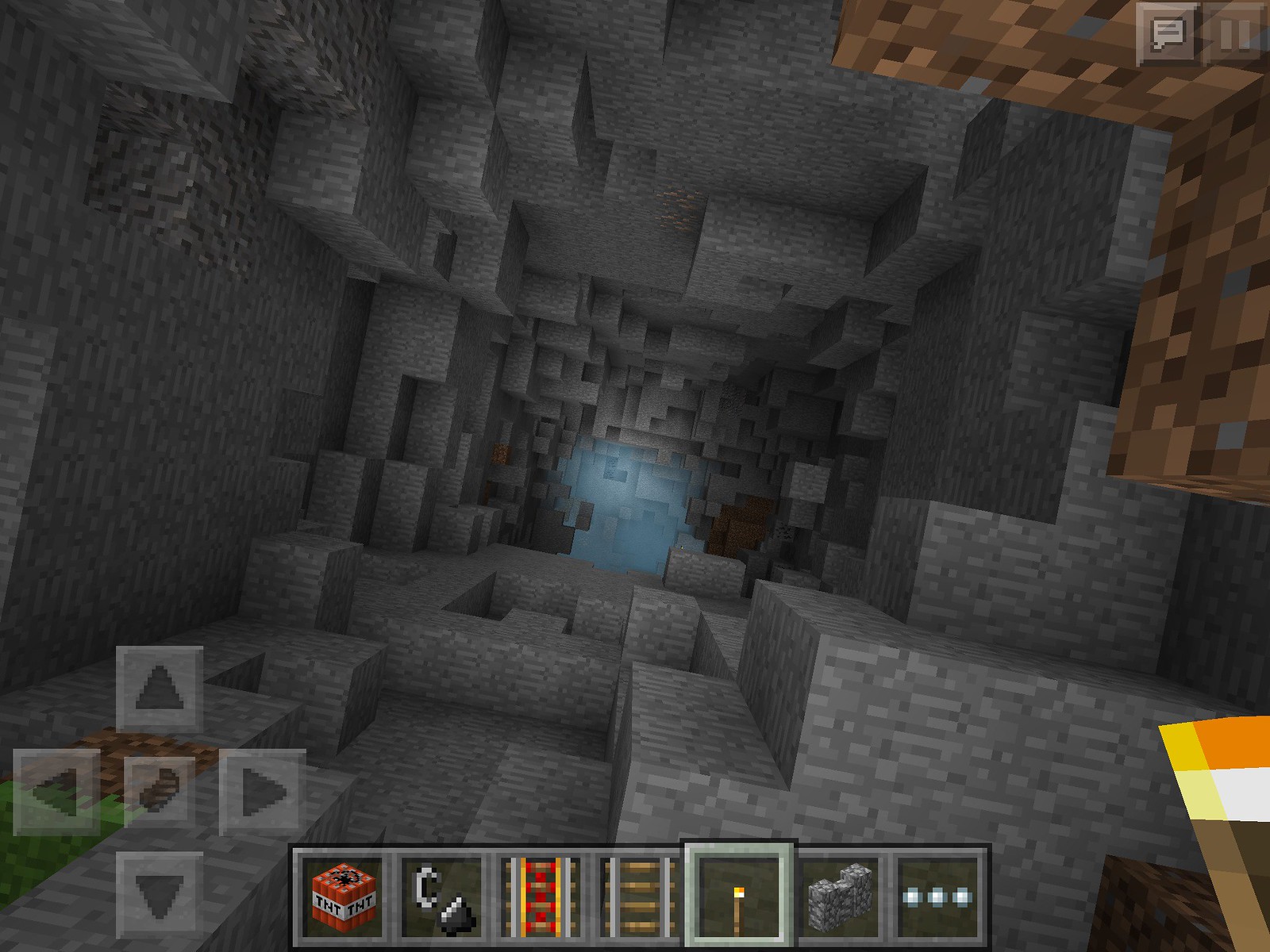The image depicts a screenshot from a video game, likely Minecraft, showing the player standing at the edge of a vast, pixelated hole. The hole itself is composed of various gray rectangular and square blocks resembling bricks, with a mix of light gray, medium gray, and dark gray tones creating a complex, three-dimensional, maze-like structure. In the upper right corner, part of the wall features shades of brown dirt, contrasted against the predominantly gray bricks. The bottom of the hole contains water, adding to the sense of depth. Along the bottom of the screen, a cross-shaped navigation interface with arrows pointing north, east, south, and west is visible on the left, while an item toolbar spans the center, displaying icons including TNT and other unidentifiable items. The overall scene is dimly lit, with some light gray areas suggesting openings or reflective surfaces, further enhancing the intricate and immersive nature of the virtual environment.